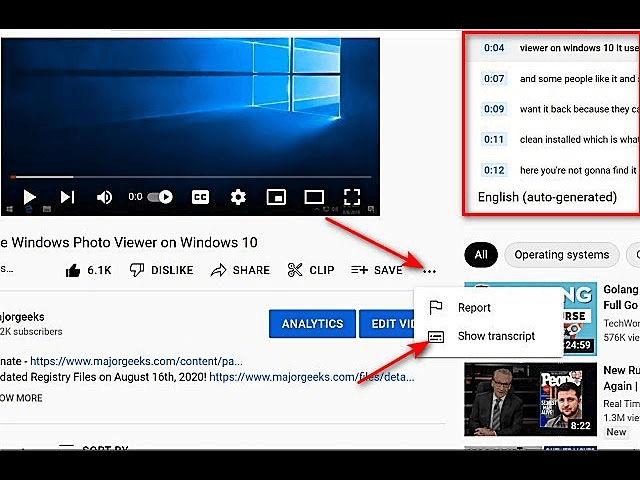This screenshot captures a section of a YouTube page, primarily featuring the interface of a video titled "Windows Photo Viewer on Windows 10". In the top left corner, part of the video player is visible, displaying a black and blue window screen along with the usual playback controls—play/pause, volume, closed captioning, and other settings—positioned at the bottom.

Directly below the video, the title "Windows Photo Viewer on Windows 10" is prominently displayed. Beneath the title, the familiar YouTube action buttons for liking, disliking, sharing, clipping, and saving the video are neatly arranged. Further down, there is information about the YouTube profile associated with the video, including various links.

Highlighted by red arrows are important features: three dots indicating additional options, and another red arrow pointing to a pop-up window with options for "Report" and "Show Transcript".

In the bottom right section of the screenshot, thumbnails for other recommended YouTube videos can be seen, facilitating further engagement. Meanwhile, in the top right, a red box captures snippets of the video's transcript. This box displays several blue rectangles marking timestamps (e.g., 4, 7, 9, 11, and 12 seconds), accompanied by corresponding segments of the transcript in black font.